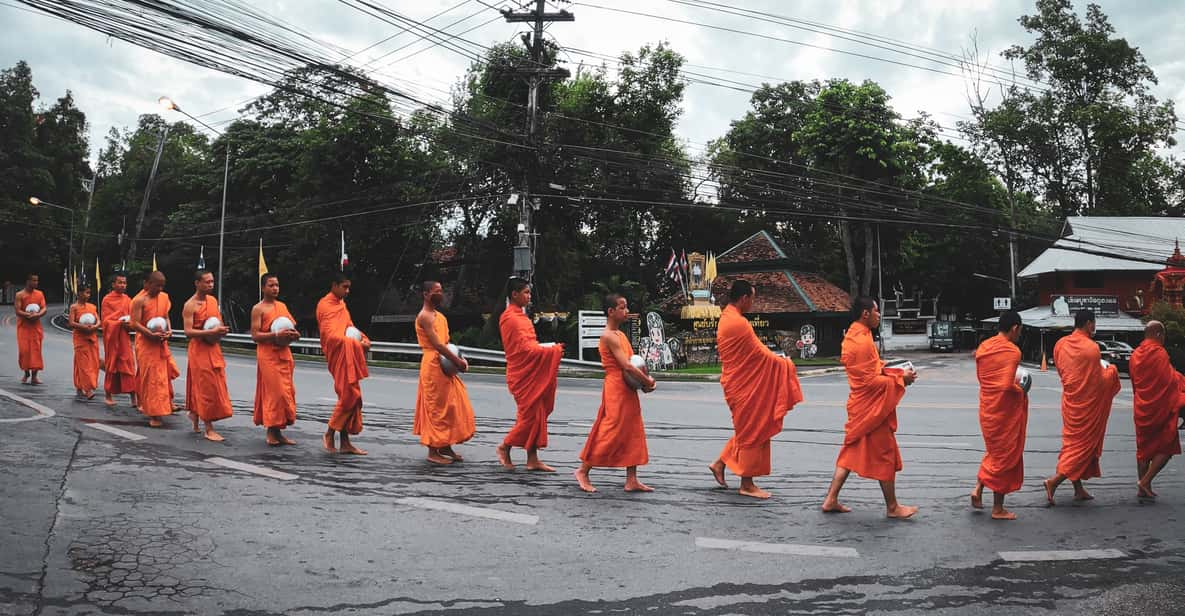This color photograph captures a serene procession of around fifteen Tibetan Buddhist monks walking single file down a gray, possibly rain-dampened street in a small town. Clad in various shades of bright orange robes that wrap around their bodies, some monks have their arms exposed, while others are covered completely. Each monk, distinguished by their close-cropped hair and darker skin, is barefoot and reverently carries a round white bowl clutched to their stomachs. 

The background is a mix of urban and natural elements; we see several buildings or shops, some with brown or white roofs, which suggest local businesses perhaps even restaurants. Overhead, there are numerous electrical wires and power lines crisscrossing the cloudy, greyish sky with tiny patches of blue. Tall, greenish-black trees add to the scenic backdrop, and yellow flags can be spotted fluttering just above the monks' heads on the left side of the image. The composition of the monks in their vibrant robes against the overcast, muted surroundings creates a striking visual contrast, emphasizing their tranquil presence and the ritualistic nature of their walk down the dotted-line pavement.